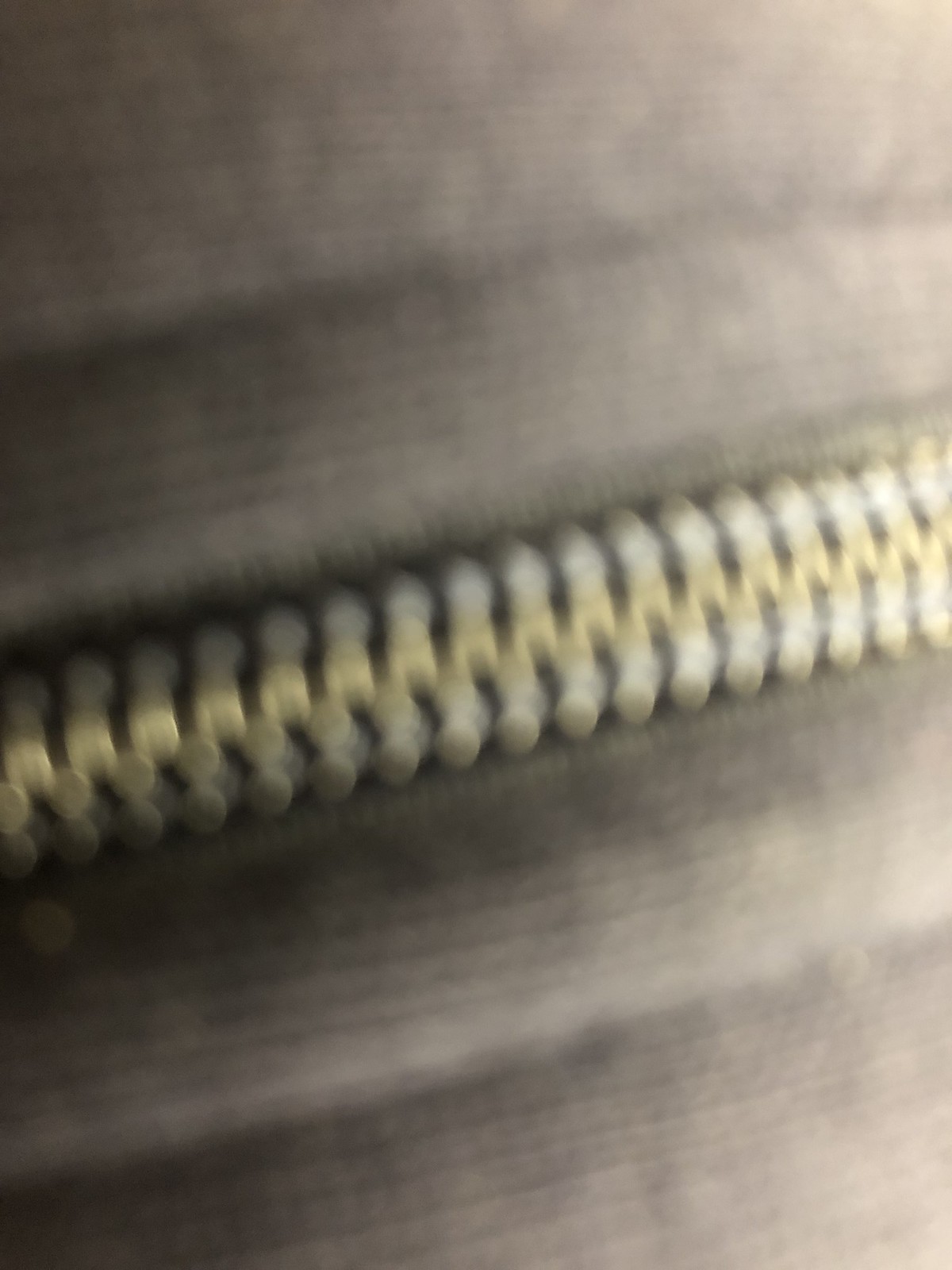This is a close-up, albeit blurry, photo of a zipper on what appears to be a knitted, zip-up sweatshirt. The zipper, oriented horizontally from left to right, features a silver outer edge with a brass-colored center. The knit material of the garment is gray. The overall image lacks clarity due to the blurriness and extreme zoom.